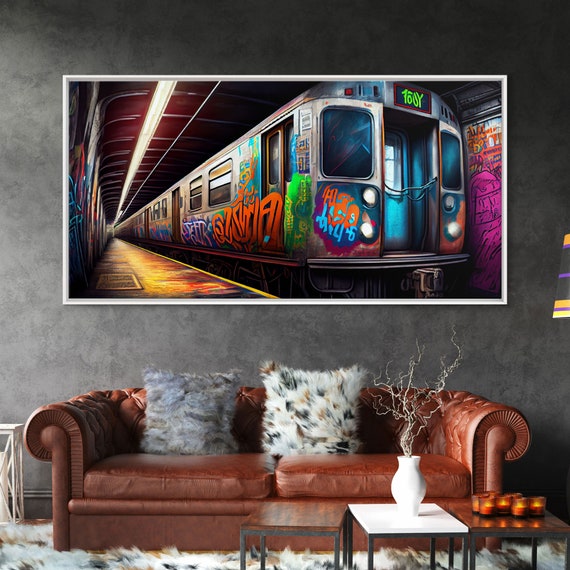This image depicts a modern living room dominated by a light brown leather couch adorned with two furry pillows, a gray one on the left and a white one on the right. Above the couch hangs a vibrant painting of a silver subway car, heavily tagged with neon-colored graffiti in hues of blue, green, orange, and pink. The artwork, set against gray walls, showcases the subway train facing the viewer with no passengers and a light strip crossing the ceiling of the subway car. The floor of the room is covered by a white and black furry rug. In front of the couch are three small coffee tables; the central white table holds a white vase with what appears to be a dead plant, while the darker tables on either side feature several small orange candles. The entire setting emphasizes a blend of neutral tones for the furniture and striking, colorful art for a modern aesthetic.